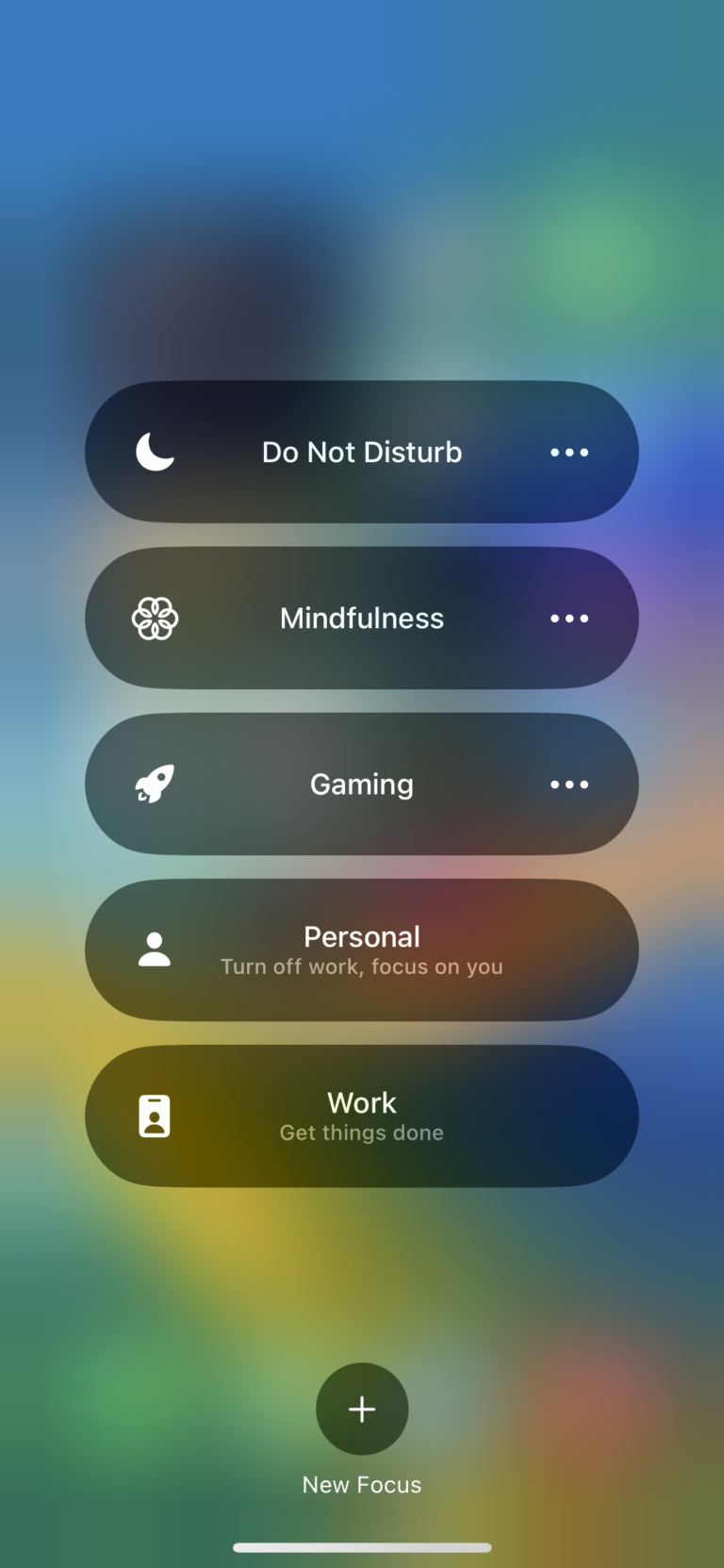The image is a screenshot, likely taken from a phone, indicated by the presence of a distinctive white line at the bottom of the screen, which typically appears on phones. The background of the screenshot is a hazy blur of colors with a gradient transition. The top section is dominated by blue, followed by patches of black, green, and white. As the colors shift downward, the middle section features shades of pink and orange, while the bottom section integrates yellow, green, white, and pink hues again.

Centrally, the screen displays five selectable options, each presented as elongated oval-shaped bars. These bars are positioned against a dark gray backdrop. The first option features a crescent moon icon and is labeled "Do Not Disturb," with an ellipsis (three dots) on the right side. The second option is marked by a flower icon and the word "Mindfulness," also accompanied by an ellipsis. The third option displays a rocket ship icon labeled "Gaming," with the same ellipsis on the right. The fourth option has an icon of a person and is labeled "Personal," with an additional subtitle underneath that says, "Turn off work, focus on you." The fifth option shows an icon representing an ID badge, labeled "Work," with a subtitle that reads, "Get things done."

All main text is rendered in a clear white font, while the subtitles use a very light white font for differentiation. Positioned centrally at the bottom of the screen is a gray circle with a plus sign in the center. Directly beneath this circle are the words "New Focus."